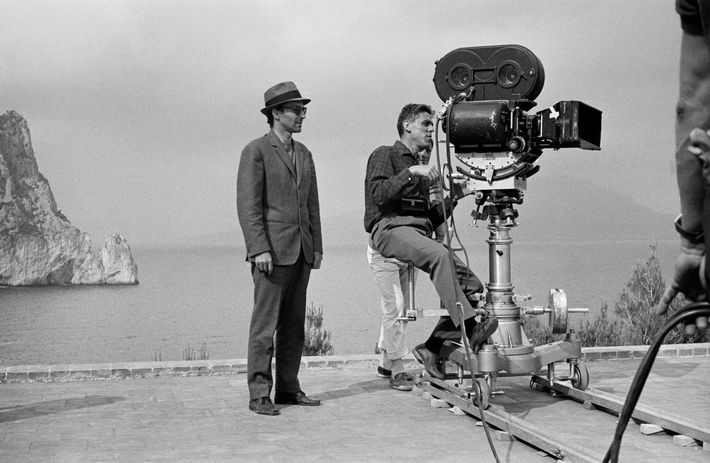This black and white photograph captures what appears to be a movie set styled to evoke the 1980s, suggested by the fashion and general ambiance. Central to the scene are two men: one is seated behind a camera positioned on a rolling platform, seemingly engrossed in his task. The second man stands nearby, exuding a cool demeanor with his dark sunglasses and brimmed hat. He is smartly dressed in a suit, adding to the retro vibe. In the background, a portion of the set depicts a small grassy hill, reinforcing the picture's vintage aesthetic.